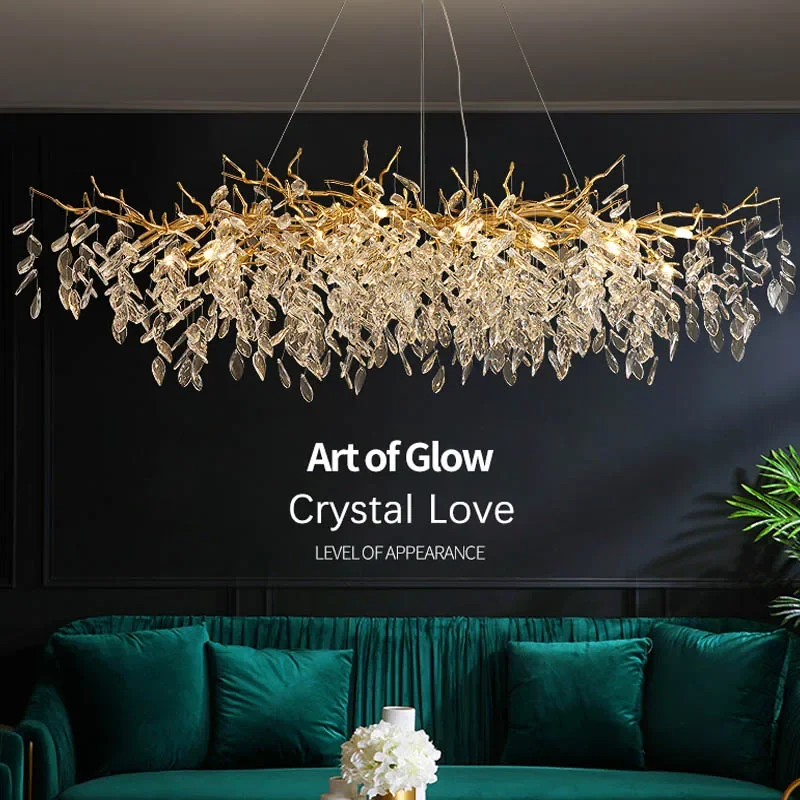The photograph captures an intricate chandelier hanging from the ceiling, supported by four wires. This unique chandelier resembles a cluster of light brown, stick-like branches adorned with numerous clear and goldish-brown crystal leaves that are lit from within, creating a stunning visual effect. The chandelier is horizontally oriented, stretching from the left to the right side of the image, unlike traditional circular chandeliers.

Below the chandelier is a green couch with four green pillows, positioned against a black wall. In front of the sofa is a white floral arrangement in a golden vase, though the vase is cut off at the top. A slender-leaved plant is partially visible on the right side of the image, and the ceiling is a contrasting beige or off-white color. Text overlay in the middle of the photograph reads "Art of Glow, Crystal Love, Level of Appearance." The scene exudes a blend of elegance and chaos, highlighted by the ornate chandelier and the meticulous arrangement of furniture and decor.